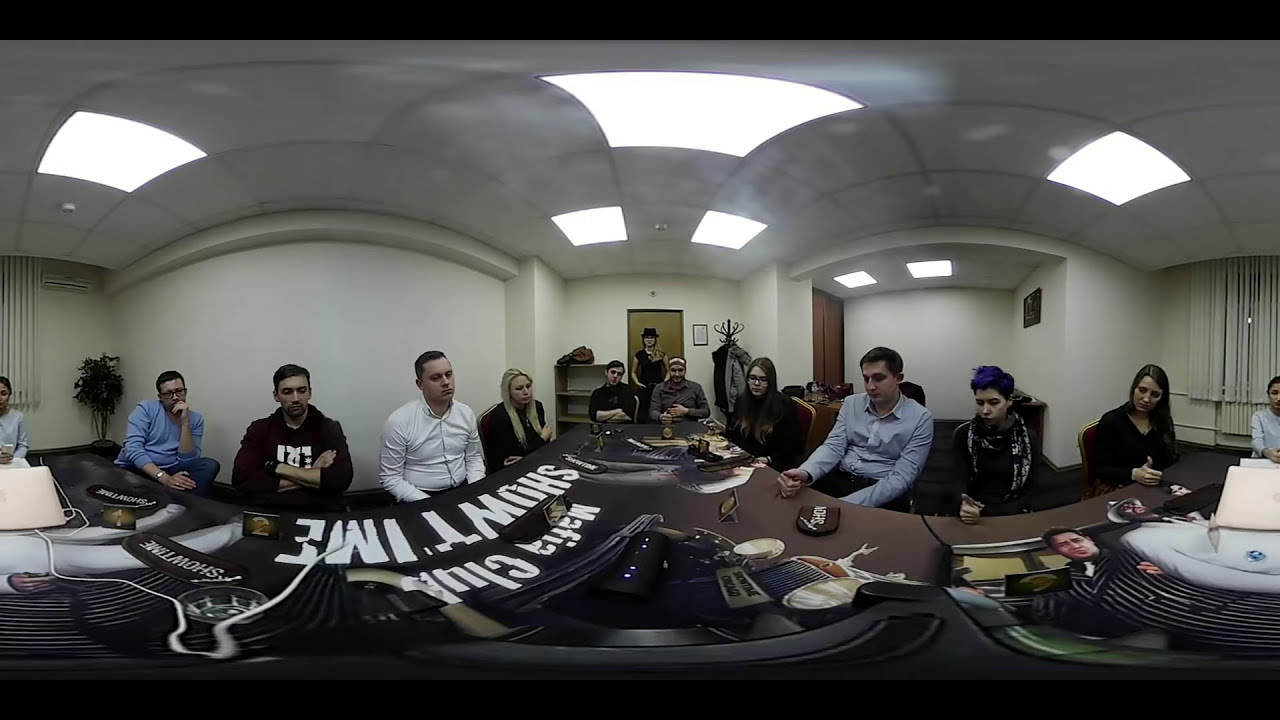This indoor photograph captures a somewhat distorted, wide-angled view of a meeting room, possibly taken with a webcam as evidenced by the curved ceiling and walls. A diverse group of men and women, dressed in casual to business casual attire, are seated around a long brown table filled with various items, likely papers and other office materials. The table stretches across the foreground, framed by white walls and a tile ceiling lined with fluorescent lights. On the left side, notable figures include a man in a blue shirt with glasses, a man in a black sweatshirt with a white design, and a man in a white shirt. A woman with long blonde hair and a black shirt is seated further down. In the background, several men and a woman in a dark shirt and glasses can be seen, along with a man in a blue shirt with dark hair, and a woman with blue hair on the far right. Behind them are two brown doors and various office furnishings like a coat rack and a shelf. A banner on the table hints at the context, displaying the words "Mafia Club" and "Showtime."